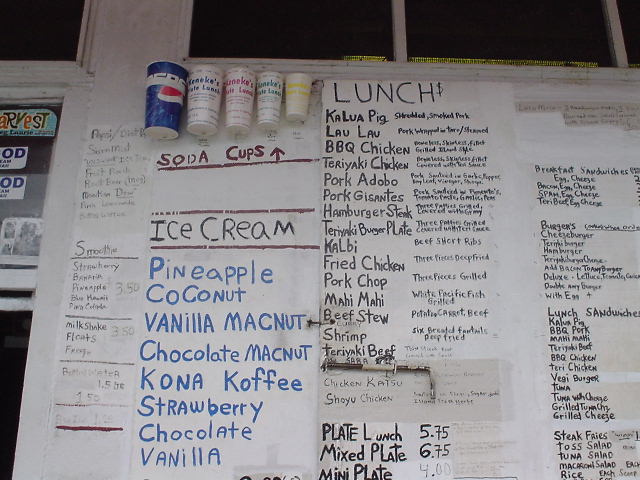This image depicts a bustling lunch truck menu, vividly handwritten, exuding a rustic, homemade charm. 

In the upper left corner, a row of soda cups is illustrated with a corresponding label "Soda Cups" followed by an arrow pointing upwards. The cups are arranged in descending order of size, starting with a large Pepsi cup on the left, shrinking to increasingly smaller sizes.

Directly beneath this section, the menu features a list of ice cream flavors written in black lettering. It reads "Ice Cream," followed by a variety of flavors in blue text: pineapple, coconut, vanilla, macadamia nut, chocolate, macadamia nut again, coffee, strawberry, chocolate again, and vanilla once more.

Shifting focus to the right, the top categorizes "Lunch" with a dollar sign symbolizing pricing. Below, a column details various lunch options with their respective descriptions:
- Kalua pig (shredded smoked pork)
- Lawa Lawa (pork wrapped in taro leaves)
- BBQ chicken 
- Teriyaki chicken 
- Adobo 
- Pork Gigantes 
- Hamburger steak 
- Teriyaki burger plate 
- Colby 
- Fried chicken 
- Pork chop 
- Mahi Mahi 
- Beef stew 
- Shrimp 
- Teriyaki beef.

Lower on this section, additional dishes include:
- Chicken katsu
- Shoyu chicken

The menu also offers various plate lunches:
- Plate lunch for $5.75
- Mixed plate for $6.75
- Mini plate for $4.40

Among sandwich options, labeled "Backflip Sandwiches", there are choices like:
- Egg cheese
- Bacon egg cheese
- Spam egg cheese
- Teri beef egg cheese

Beneath the sandwiches, the burgers' section includes:
- Cheeseburger
- Teriyaki burger
- Hamburger
- An additional unreadable type of teriyaki.
The menu highlights customizable options, allowing customers to add bacon to any burger or make it deluxe by doubling any burger with egg.

Lastly, additional entrees and sides are listed, including:
- Kalua pork
- BBQ pork
- Mahi Mahi 
- Teriyaki beef
- BBQ chicken
- Teriyaki chicken
- Veggie burger
- Tuna
- Tuna with cheese
- Grilled tuna cheese
- Grilled cheese
- Steak fries
- Tossed salad
- Tuna salad
- Macaroni salad
- Rice

Essence of a nose-to-tail dining experience encapsulated within this lively menu, perfect for those seeking a diverse and satisfying meal.